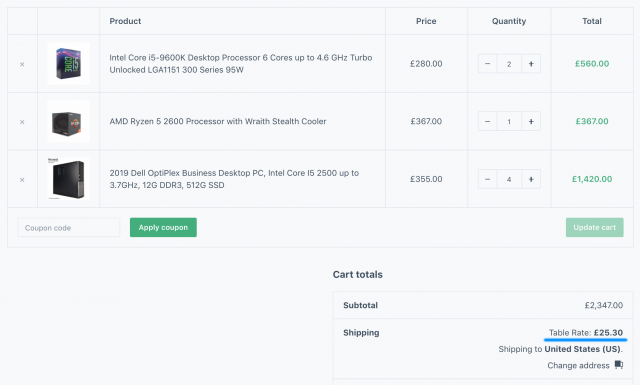A user is browsing an online store to purchase computer components, seemingly for a custom-built PC project. Their shopping cart displays three distinct items: two Intel Core i5-9600K desktop processors (six cores, up to 4.6 GHz), one AMD Ryzen 5 2600 processor, and four 2019 Dell Optiplex business desktop PCs (Intel Core i5-2500, up to 3.7 GHz). Despite the mix of components that don't typically go together, the user has selected these items for a combined subtotal of £2,347. The order is set for international shipping to the United States.